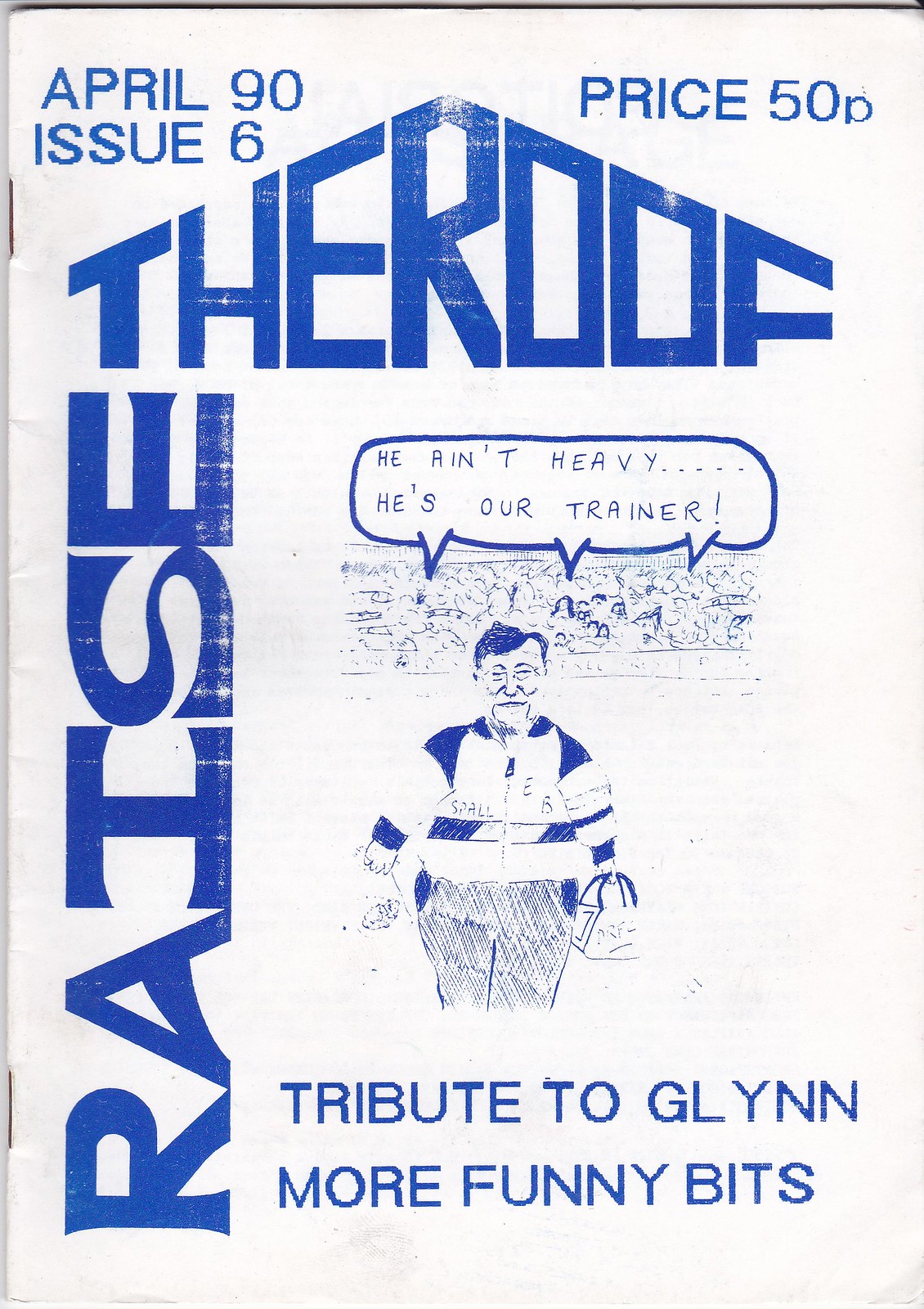This image is a vertically aligned, rectangular poster resembling a booklet cover with a light grayish-white background, annotated in royal blue ink. Along the top edge, it reads "April 90," followed by "Issue 6" and "Price 50p." The phrase "Raise the Roof" is cleverly integrated with "Raise" running vertically from bottom to top on the left side, and "The Roof" horizontally across the top right. The focal point of the poster is a cartoon-style drawing in the center, featuring a heavyset man with short, combed-over hair and glasses, wearing a striped shirt and pants, holding a small bag. Behind him is a crowd, with a speech bubble that states, "He ain't heavy, he's our trainer." At the bottom, the text "Tribute to Glyn," along with "More funny bits," completes the design.